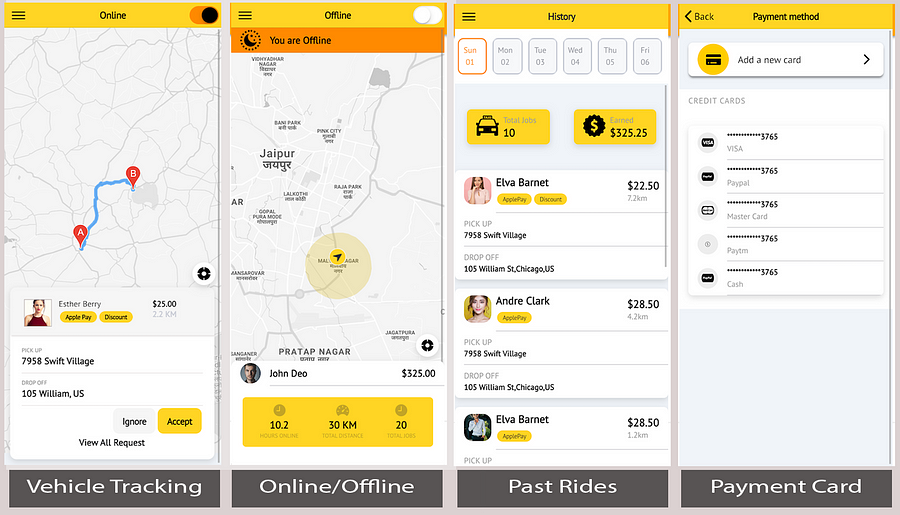This series of screen captures appears to showcase various functionalities and interfaces of the same ride-sharing application, dominated by hues of orange, gold, black, white, and gray.

The initial screen features a conspicuous gold bar adorned with three black lines next to an orange circle. Below this, a map is depicted with markers labeled 'Point A' and 'Point B,' connected by a blue line. The screen displays the name "Esther Berry," an option for "Apple Pay or Checkout" marked at $25, and an image of a woman. Following this, it lists an address as "7958 Swift Village" and another as "105 William U.S." There are options for pickup and drop-off at these locations, alongside buttons labeled "Ignore," "Accept," and "View All Requests." At the bottom, "Vehicle Tracking" is mentioned in gray and white.

The next screen features a gold and black banner indicating "Offline" with a smaller orange notification and a moon icon stating, "You are offline." Below this, a map icon with a gold circle is visible, showing information for an individual named "John Dio" worth $325 U.S. A gold box displays "10.2, 30 KM, and 20," and "Online/Offline" is written in gray and white.

Following this, a history screen provides a detailed breakdown of days, marked by gold and black headings, including Sunday the 1st to Friday the 6th. It highlights total jobs completed, reflecting 10, and earnings of $325.25. Information about 'Elva Barnett,' displayed with a woman’s image in pink, includes two gold boxes labeled "2250," with pickup and drop-off details between "7958 Swift Village" and "105 Williams Street, Chicago, U.S." Similarly, details for 'Andre Clark' show 2850, accompanied by the same addresses.

A section termed "Past Rides" encapsulates previous journey details, followed by a payment method screen. This screen in gray and black prompts with "Payment Method Back" and has a white box allowing new card additions, adorned with a gold and black card logo. Listed payment options include "Visa ending in 3765," "PayPal," and "MasterCard." At the bottom, it concludes with "Payment Card," in gray and white. 

This detailed series of screens collectively represents components of user interactions within the ride-sharing application, focusing on navigational, financial, and historical aspects.